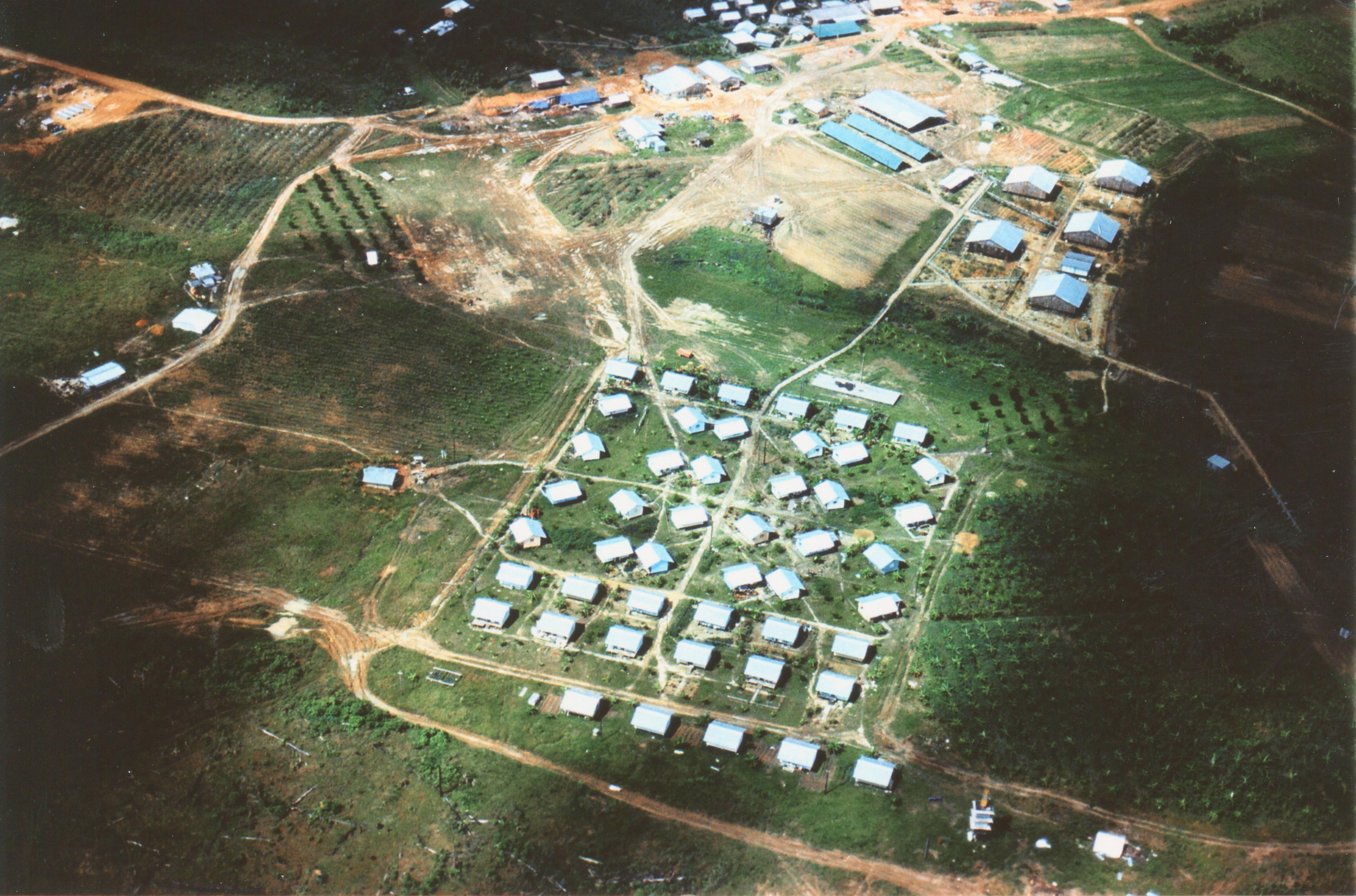This aerial photograph captures a vast rural landscape interspersed with various structures and fields. The central focus is a cluster of approximately 30 closely-packed buildings with silver and white roofs, arranged in a square pattern with dirt roads weaving between them, giving the appearance of a small neighborhood or tightly knit community. Above this central area, towards the upper right corner, are longer, rectangular buildings with silver roofs, suggesting agricultural or industrial purposes, possibly farm or factory-related structures like chicken coops or large barns. Surrounding these buildings are extensive green fields of various shapes, some appearing to be orchards, interspersed with brown dirt roads. The image, likely taken from an airplane, shows a structured yet rural environment where small developments punctuate the expansive fields, hinting at a blend of agricultural activity and residential life.